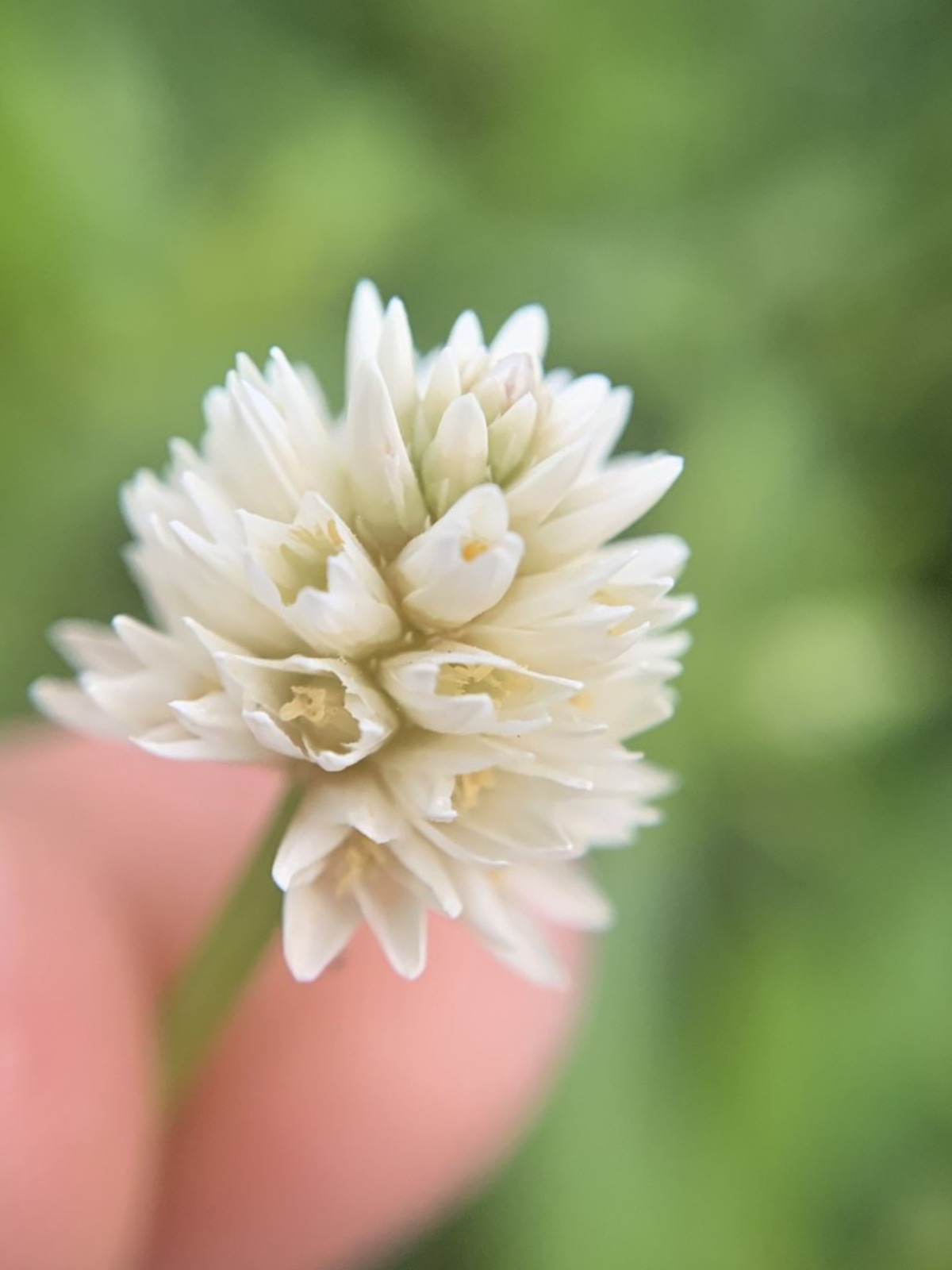This color photograph, in portrait orientation, captures a close-up, outdoor view of a white clover flower during the daytime. The photograph, approximately six inches high by four inches wide, prominently features a single cluster of small, white, conical-shaped petals forming a rounded head on a light green stem. The focus is sharply on the clover's blossoms, which have elongated tips and cream-yellow stamens within. In the lower left-hand corner, slightly blurred, are the tips of a person's fingers of Caucasian descent holding the stem. The background consists of a green, blurred-out field, possibly featuring additional foliage and a faint patch of pink. The image uses a shallow depth of field, emphasizing the intricate details of the clover blossom while keeping other elements softly out of focus.